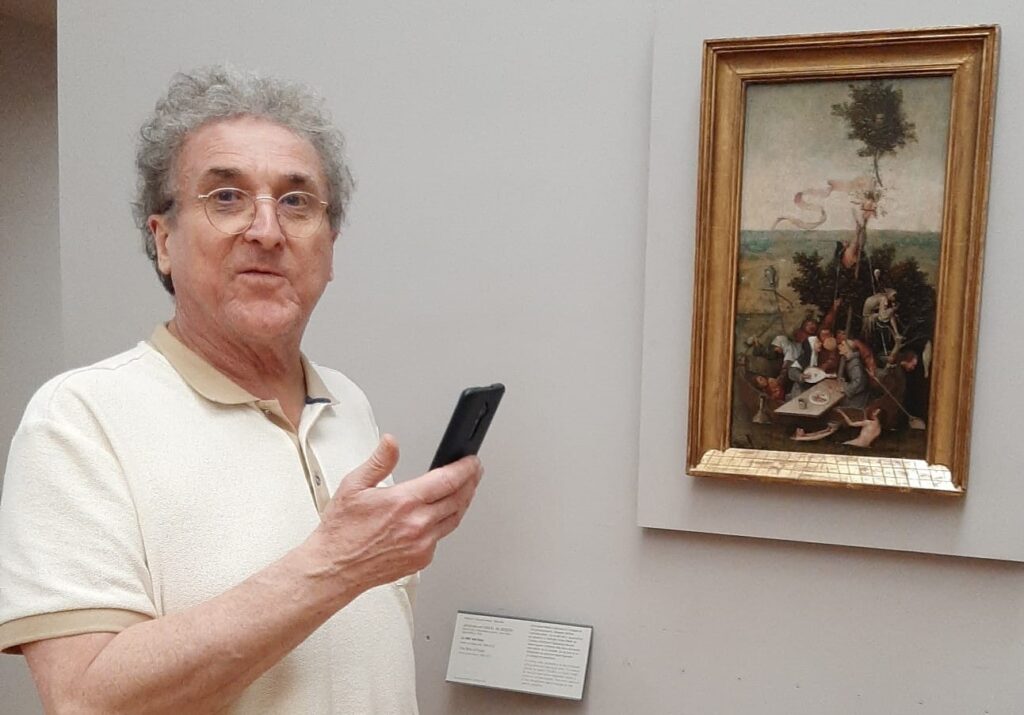An older Caucasian man, estimated to be around 65 to 70 years old, with gray, slightly curly hair and glasses, is standing and looking directly at the camera with a neutral expression. He is wearing a short-sleeved white shirt with tan-colored accents on the collar and sleeve ends. In his right hand, he holds a black smartphone, which appears to potentially be an Android device, indicated by the centrally-placed camera on its back. The man stands in front of a very light coffee-colored wall, which serves as the backdrop for the scene. To his right, there is a gold-framed picture that appears to be an intricate 16th-century style painting depicting a gathering of people around a dining table, possibly with a tree and ribbons, although the details are hard to discern. Below the painting, towards the bottom of the wall, is a small white placard with black text, suggesting information about the artwork, though the specifics of the writing are not legible.